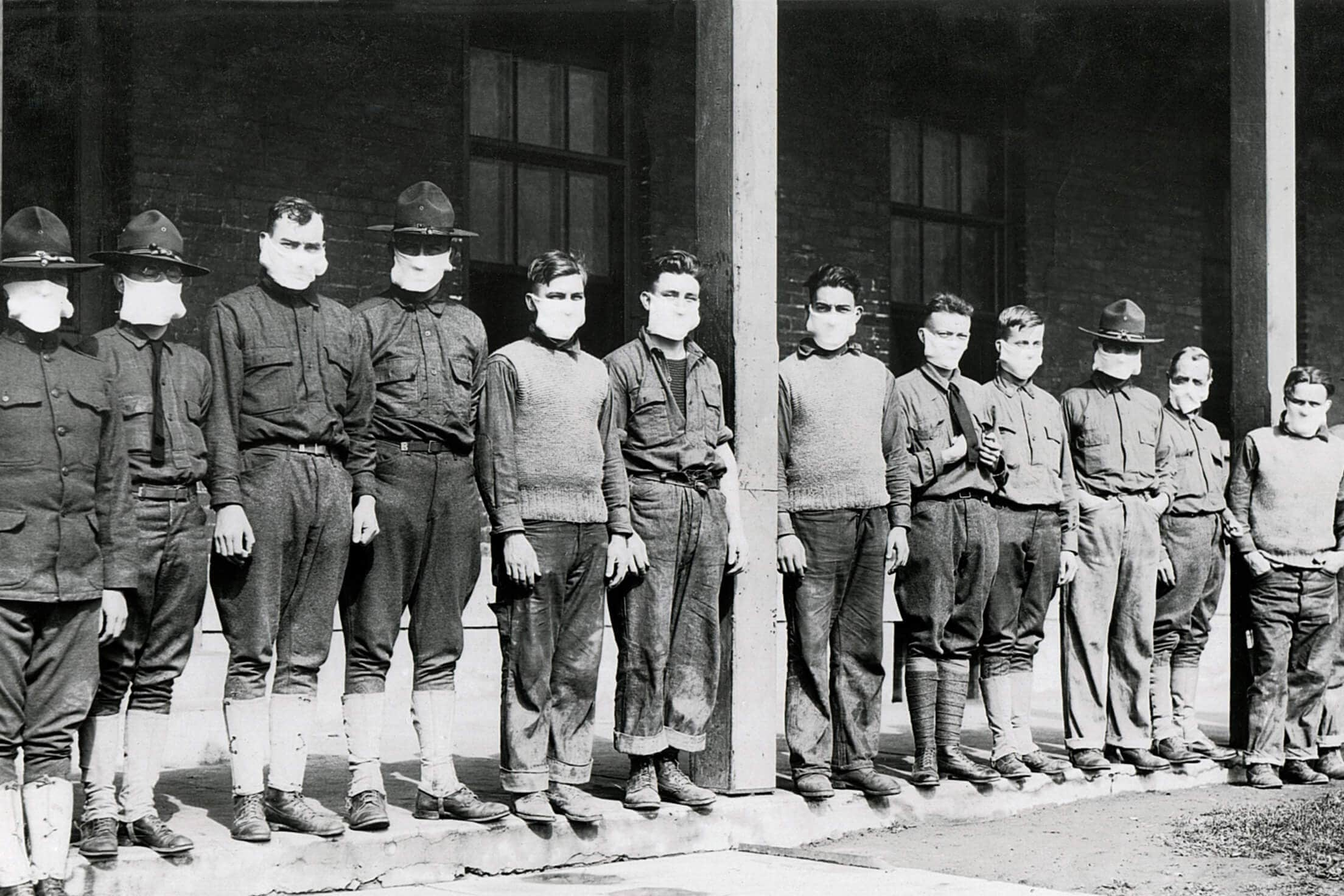This black-and-white photograph appears to be from an old era and depicts a group of approximately ten men standing side by side in a straight line on the patio of a large brick building with black-paned windows. The men are outfitted in military or possibly ranger attire, characterized by dark trousers, button-up shirts, boots, and various hats including sheriff-like and ranger-style hats. Additionally, some are dressed in sweater vests and ties, while others have leg wraps around their shins. Each man is wearing a white mask over his nose and mouth. The building is supported by two visible posts, and a gravel or dirt field stretches out ahead of them. They stand at attention, suggesting a formal or disciplined setting.